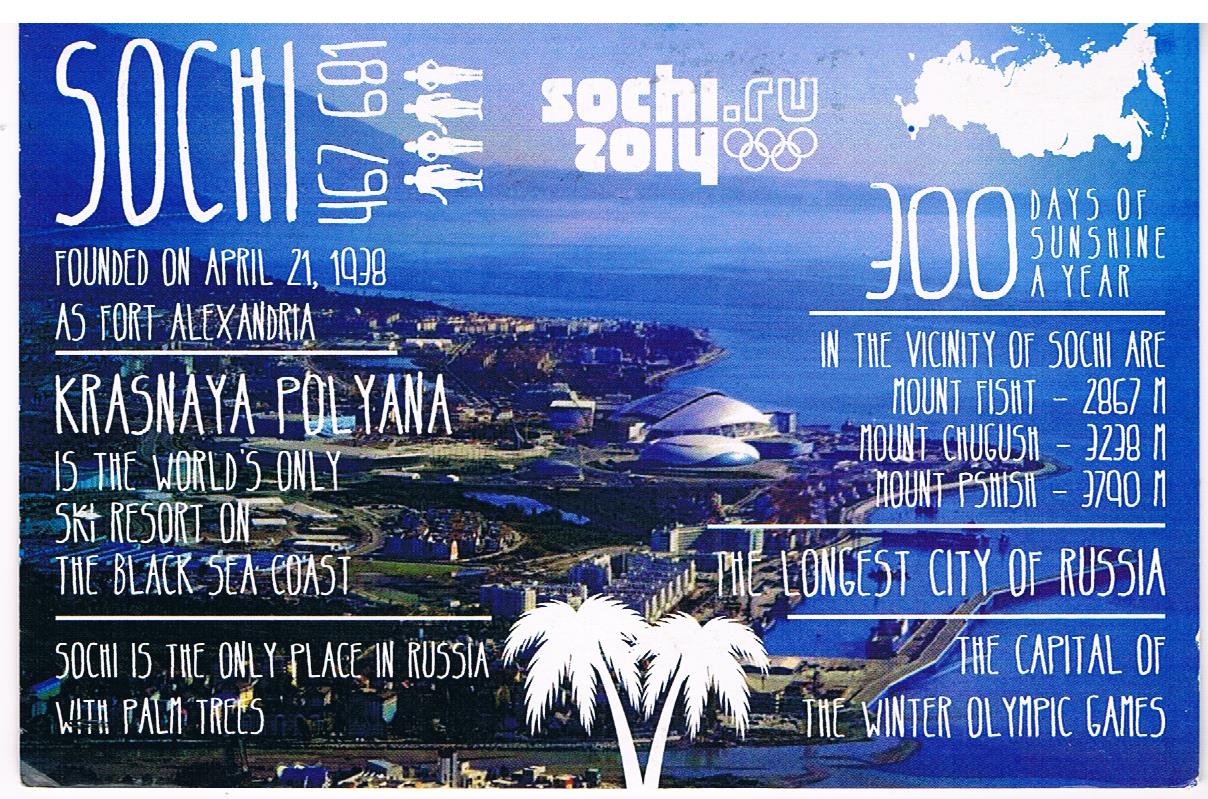The image is an informational poster or card about Sochi, a city in Russia. It features an aerial view of the city with the ocean to the right and the sky at the top. The background includes various shades of blue, white, gray, green, tan, and brown. Overlaying this scenic backdrop is a mix of text and images, providing rich details about Sochi. 

Prominently displayed in white print are key facts, including: "Sochi, 467,681 people. Sochi.RU Zoli," alongside the Olympic insignia. It highlights that Sochi enjoys 300 days of sunshine per year and was founded on April 21st, 1938, originally as Fort Alexandria. The text proudly states that Sochi is the only place in Russia with palm trees and features the Krasnaya Polyana, the world's only ski resort on the Black Sea coast.

Additional geographical information points out nearby mountain peaks: Mount Fisht at 2,867 meters, Mount Khugush at 3,238 meters, and Mount Ptsitsi at 3,790 meters. The card also notes that Sochi is the longest city in Russia and served as the capital for the Winter Olympic Games. In the foreground, white palm trees and a map in white are positioned on the right, while a cityscape near the waterfront is on the left, adding a sense of place and scale to the promotional material.